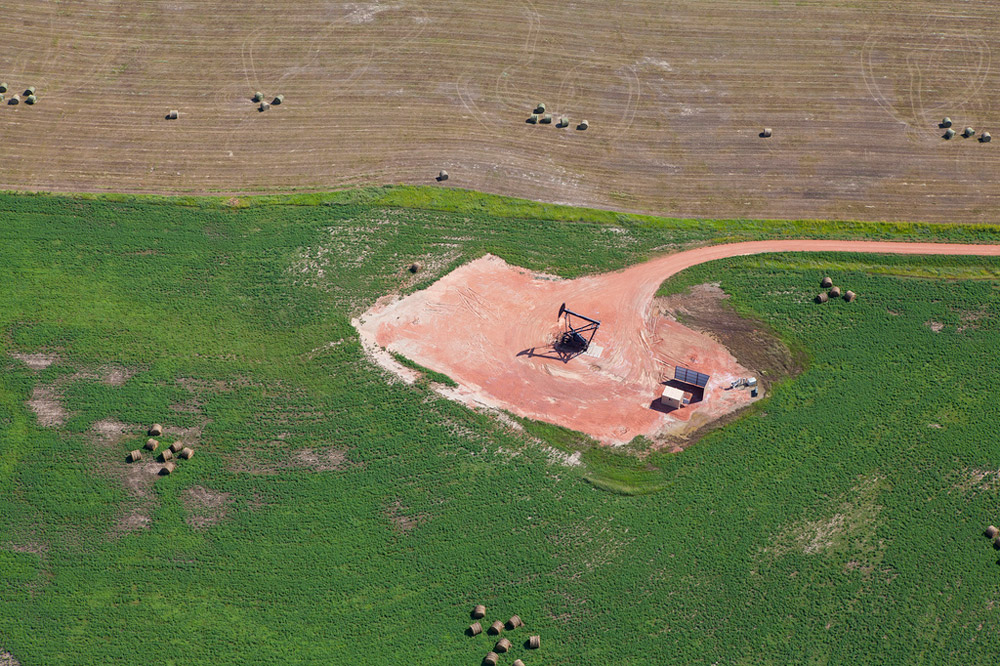An aerial photograph captures two adjacent fields dominated by green and brown hues. The upper third of the image features a recently tilled brown dirt field scattered with round hay bales, the tractor tire prints conspicuously visible around them. The lower two-thirds of the image showcases a lush, green grass field, also dotted with round hay bales that lie loose, unstacked, and strategically placed. A well-used dirt road cuts through the green field, leading to a large, square dirt patch at the center. This patch hosts a basketball hoop, sans net, suggesting some recreational use, although the structure supporting it appears jury-rigged. Nearby, towards the right corner of this patch, stands a small white building with a metal roof, and to the far right, two additional smaller buildings can be seen. The scene is completed by a black or green sign extending from the ground, adding to the rural tableau. The photograph, likely taken from a significant height, provides a comprehensive view of this agricultural and slightly industrialized landscape.